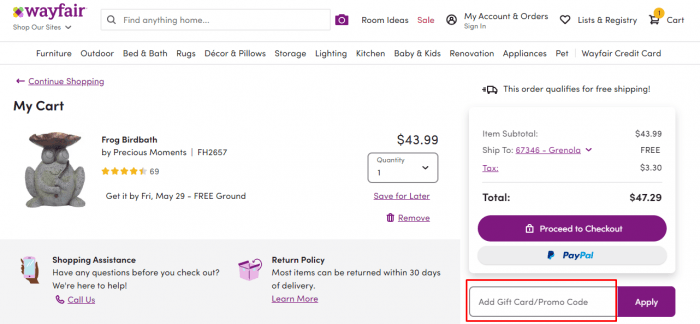The image depicts a section of the Wayfair website with a clean, white background. At the top, there is a small Wayfair logo accompanied by the name "Wayfair" in lowercase and purple letters. Below this logo is the phrase "Shop Our Sites" with a downward arrow, suggesting a dropdown menu.

To the right, there is a search bar with a magnifying glass icon, featuring the placeholder text "find anything home..." Next to the search bar is a purple camera icon. Continuing to the right, the website displays navigational options: "Ideas", "Sale" in pink, and an icon of a person's head and shoulders labeled "My Account". "Order Sign In" appears nearby, followed by a heart icon denoting "Lists & Registries". There is also a shopping cart icon containing the number '1' within a yellow circle, indicating one item in the cart.

Beneath this, a horizontal menu lists categories including Furniture, Outdoor, Bed & Bath, Rugs, Decor & Pillows, Storage, Lighting, Kitchen, Baby & Kids, Renovation, Appliances, Pet, and Wayfair Credit Card.

Further down, a purple left arrow and text "Continue Shopping" appear. On the right, there is a message stating that the order qualifies for free shipping. Below this notice, within the shopping cart section, is an order summary itemized as follows:
- A "Frog Bird Bath" priced at $43.99 (Quantity: 1), with options to "Save for Later" or "Remove".
- The total order amount is $43.99 and ships to zip code 67346 with free shipping.
- The total with tax amounts to $47.29.

Finally, options are provided to "Proceed to Checkout" or use PayPal. There is also a field to "Add Gift Card/Promo Code" bordered in red, with an adjacent "Apply" button in purple with white text.